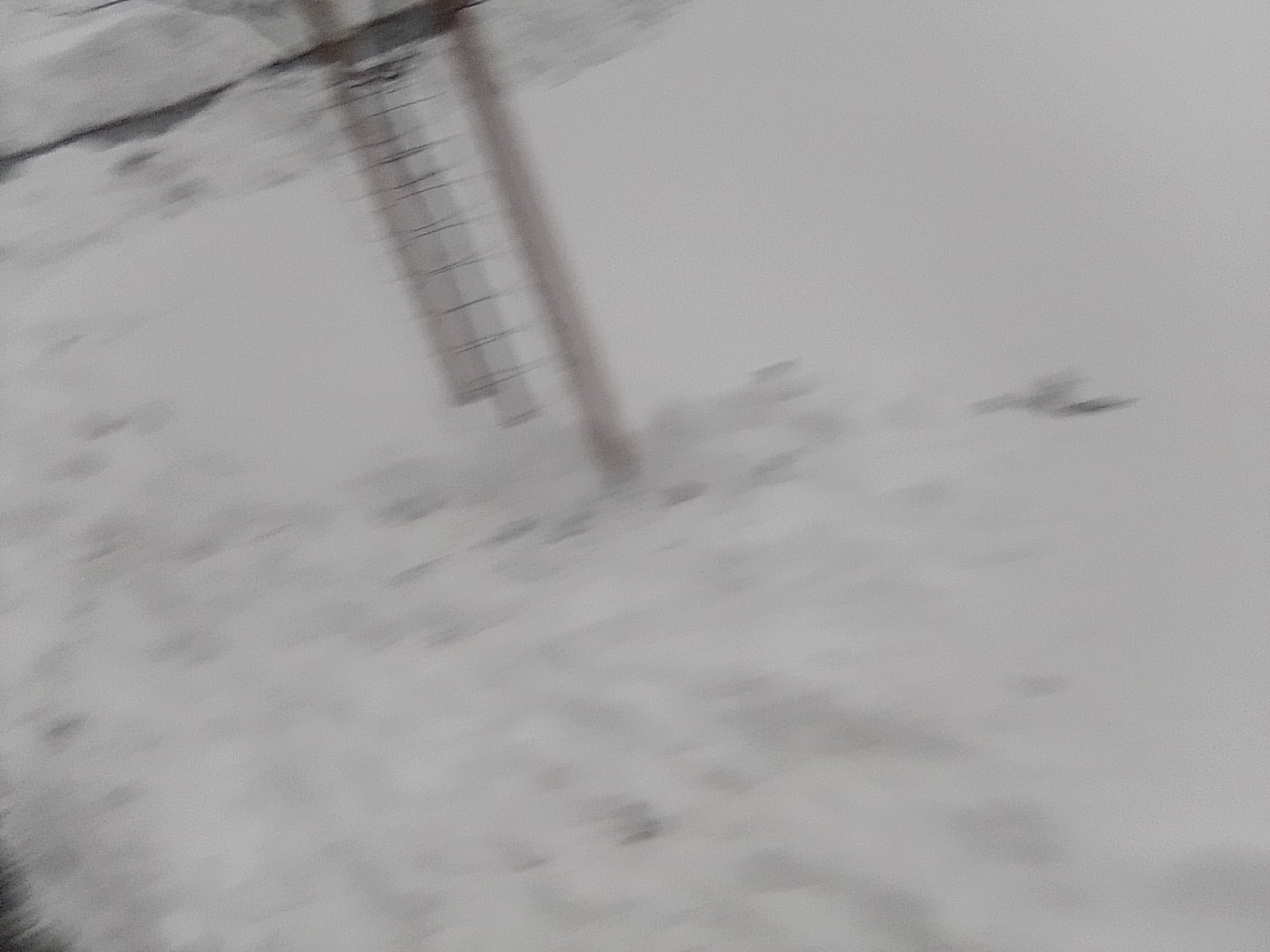The image in question is blurry and appears to have been taken while in motion, which has resulted in a lack of clarity. The overall color palette is primarily grayish, with shades of brown and darker gray interspersed throughout the scene. The image seems to depict a pale surface, potentially snow or sand, which dominates the view. Track marks, likely from footsteps, are evident, starting from the bottom left and moving towards the center, reinforcing the assumption of a snow or sand-covered ground.

From the center extending towards the upper left-hand corner, there is a discernible stick-like object with black lines emanating from it, interrupted by a dark cut near its top, whose exact nature remains unclear. The upper right corner of the photograph is smoother and evenly colored in gray, whereas the upper left corner has a more textured, ruffled appearance, possibly indicating the presence of rocks or a rugged terrain. Overall, the image elicits a sense of an outdoor setting marked by its pale, possibly snowy or sandy, landscape and ambiguous elements.